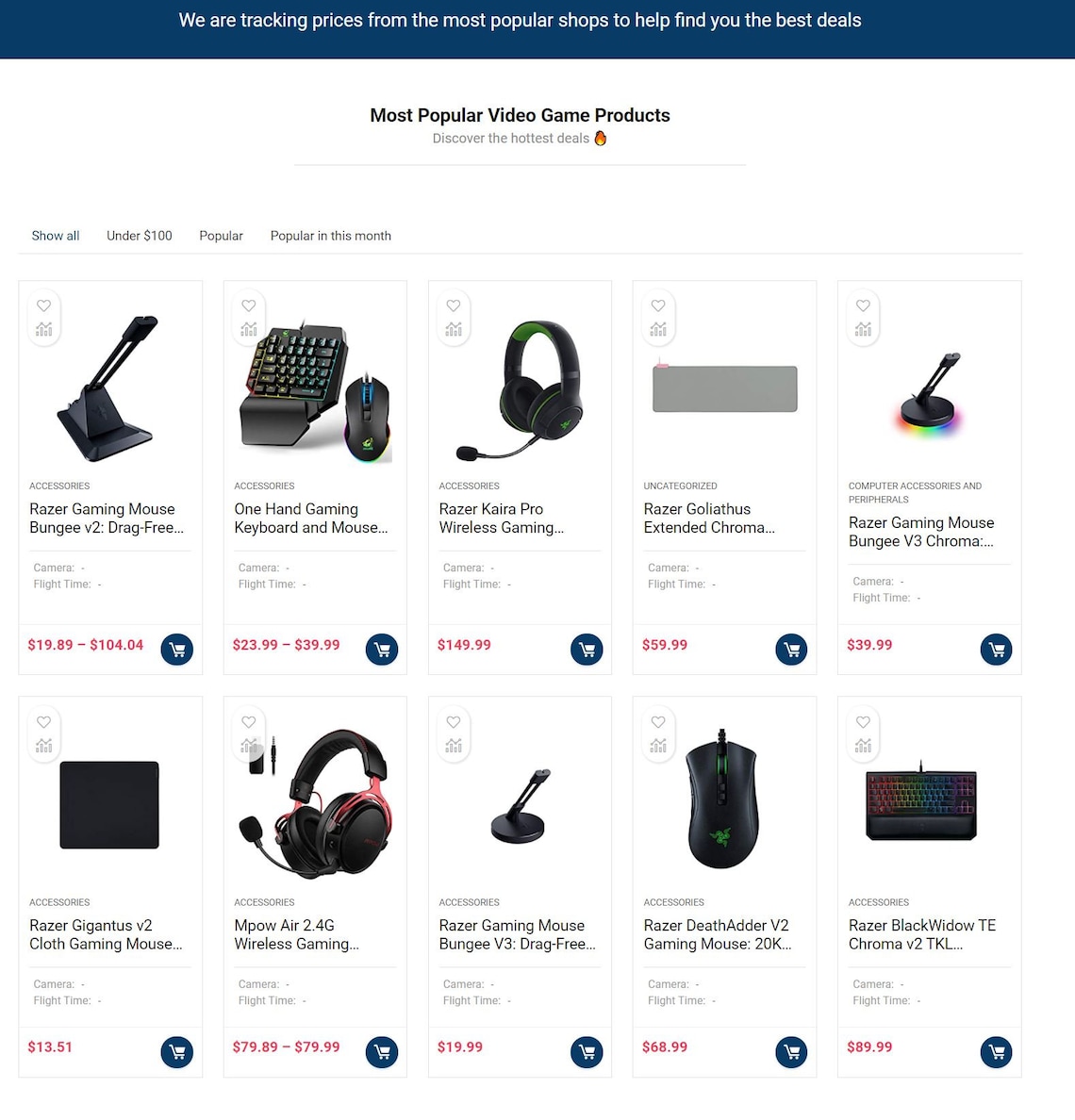This is a website for a company that specializes in providing the best deals on various products. At the top of the page, a blue banner with white lettering announces, "We are tracking prices from the most popular shops to help you find the best deals." Below this banner, centered in black text, it reads, "Most Popular Video Game Products," followed by a gray caption that states, "Discover the hottest deals," accompanied by a small flame icon.

The main section of the page displays various office and gaming products with full details:

1. **Razer Gearing Mouse Bungie V2 Drag Free**  
   - **Price Range:** $19.89 to $104.04 (Displayed in red)
   - **Features:** A high-quality mouse bungee designed for an unrestricted gaming experience.
   - **Icons:** A star and an additional, unidentified icon at the top of the image.
   - **Action:** Add to cart option available.

2. **One Hand Gaming Keyboard and Mouse**
   - **Price:** $23.99 to $39.99
   - **Features:** An ergonomic gaming keyboard and mouse set, ideal for enhancing gameplay.
   - **Action:** Add to cart option available.

3. **Razer Kyra Pro Wireless Gaming Headset**
   - **Price:** $149.99
   - **Features:** A premium wireless gaming headset that offers superior sound quality and comfort.
   - **Action:** Add to cart option available.

A total of 10 products are displayed, each featuring a clear image, a brief description, and their prices, with an option to add them to the shopping cart.